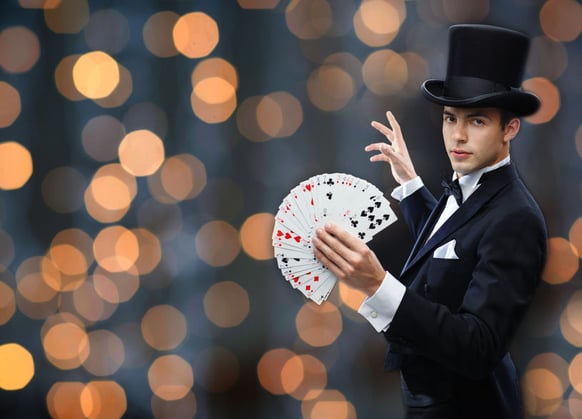The image showcases a professional magician dressed in a classic black tuxedo with a crisp white dress shirt and a black bow tie. He wears a tall black top hat with a distinctive black stripe. His left hand prominently displays a spread of black-and-white poker cards, while his right arm is raised as if mid-performance, with his right hand empty. A white handkerchief peeks out from the front left pocket of his suit jacket. The background is blurred but features a mix of light grey and warm tones, including yellow, brown, and orange light bubbles, adding a magical ambiance to the scene. The magician is looking directly into the camera, engaging the viewer with his youthful presence.